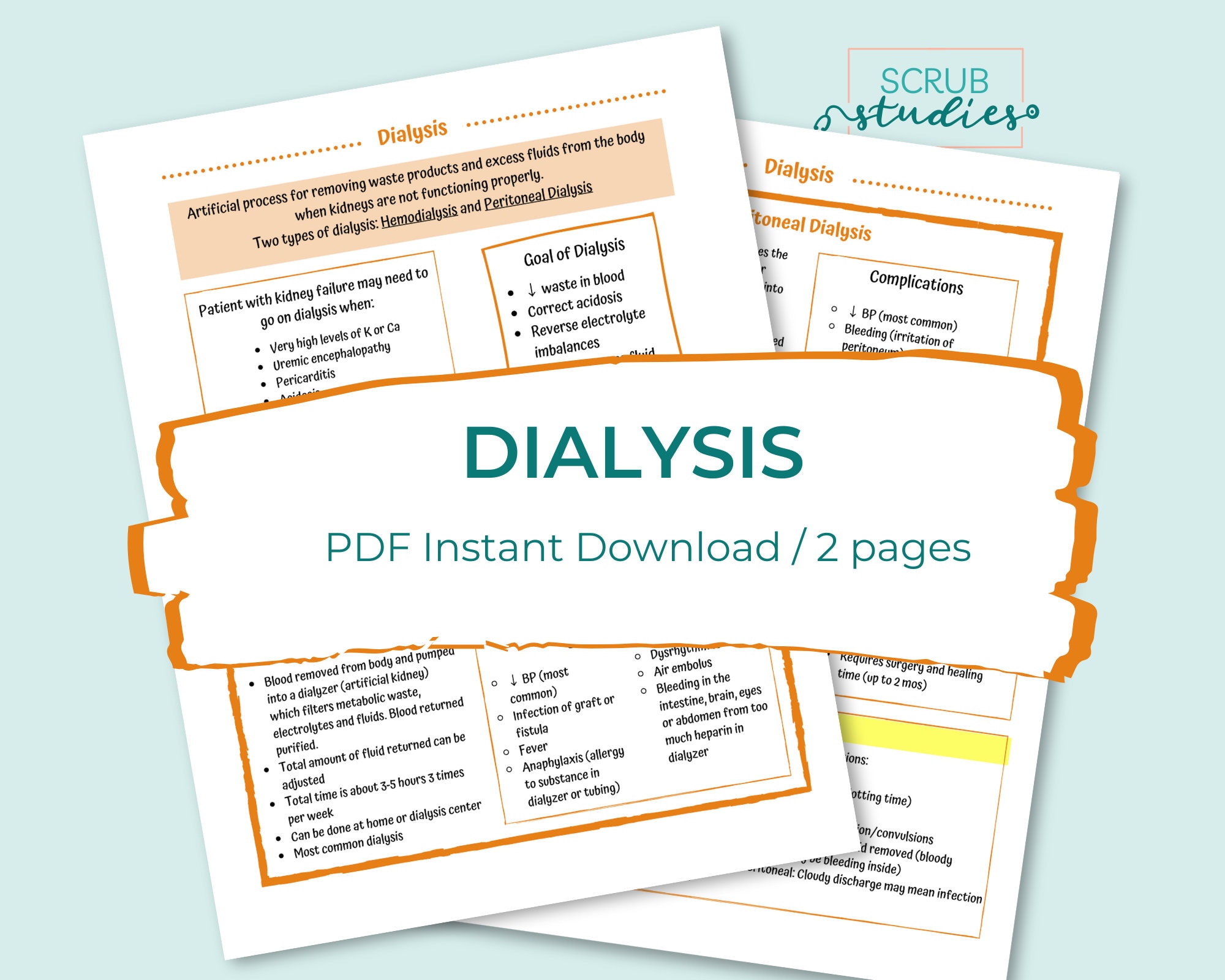Discover our meticulously crafted "Dialysis Study Guide" available as an instant PDF download. This comprehensive two-page document offers in-depth information on dialysis, perfect for both students and professionals in the medical field. The sleek design features a light teal background, with the "Scrubs Studies" logo prominently displayed in the top right corner—"Scrub" in bold teal block letters and "Studies" in elegant teal cursive, both encircled by a subtle yellow line.

Central to this guide are two intricately designed sheets overlaid on each other, detailing the fundamental aspects of dialysis. The top sheet’s title, "Dialysis," is highlighted in vibrant orange. Below, a crisp white box with an orange border accentuates the title "Dialysis" in bold teal letters, followed by "PDF instant download / two pages" in matching teal.

The guide delves into the purpose, process, and types of dialysis. Key topics include hemodialysis, peritoneal dialysis, the removal of metabolic waste, and the management of electrolyte imbalances. Detailed descriptions cover methods, benefits, and potential complications, providing a clear understanding of both the medical procedures and patient care considerations. The guide is enhanced with carefully chosen lines, boxes, and dots to organize the information for quick reference.

Ideal for quick study sessions or detailed review, this instantly downloadable PDF is an essential resource for mastering the concepts of dialysis, making it a must-have addition to any medical library.